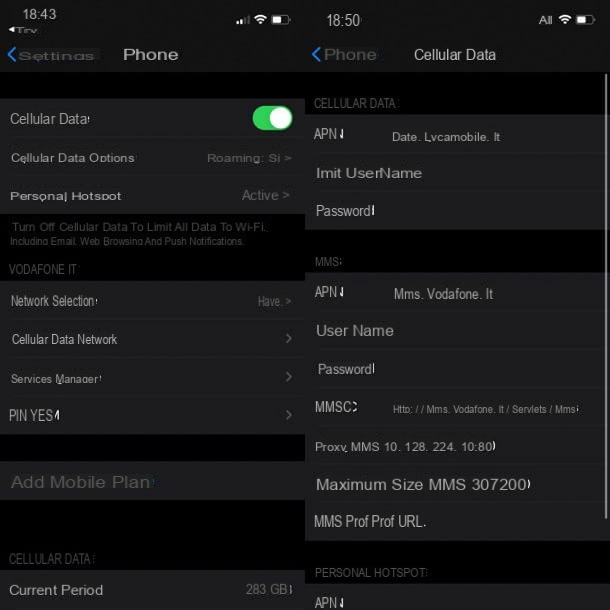Screenshot of a smartphone screen displaying two side-by-side images on a black background. The image on the left, taken at 18:43, shows the phone's settings menu, with Wi-Fi and battery icons visible at the top right. Below them, centered text indicates "Phone," and further down appears a gray, rectangular section with options labeled "Cellular Data," "Cellular Data Options," and "Personal Hotspot." The "Cellular Data" toggle is switched on. A black section below discusses turning off cellular data. Beneath that lies another gray area with options for "Network Selection," "Cellular Data Network," "Services Manager," and "SIM PIN," followed by a prompt reading "Yes, add mobile plan," and at the bottom, "Current Period."

The right image, captured at 18:50, depicts the inside of the "Cellular Data" settings. A gray box labeled "APN" followed by empty fields for "Username" and "Password" is seen at the top. Another gray box at the bottom includes fields for "APN," "Username," "Password," "MMSC," "Proxy," "MMS," "10.128.224.1080," and "Max Size," along with an "MMS Proof URL."